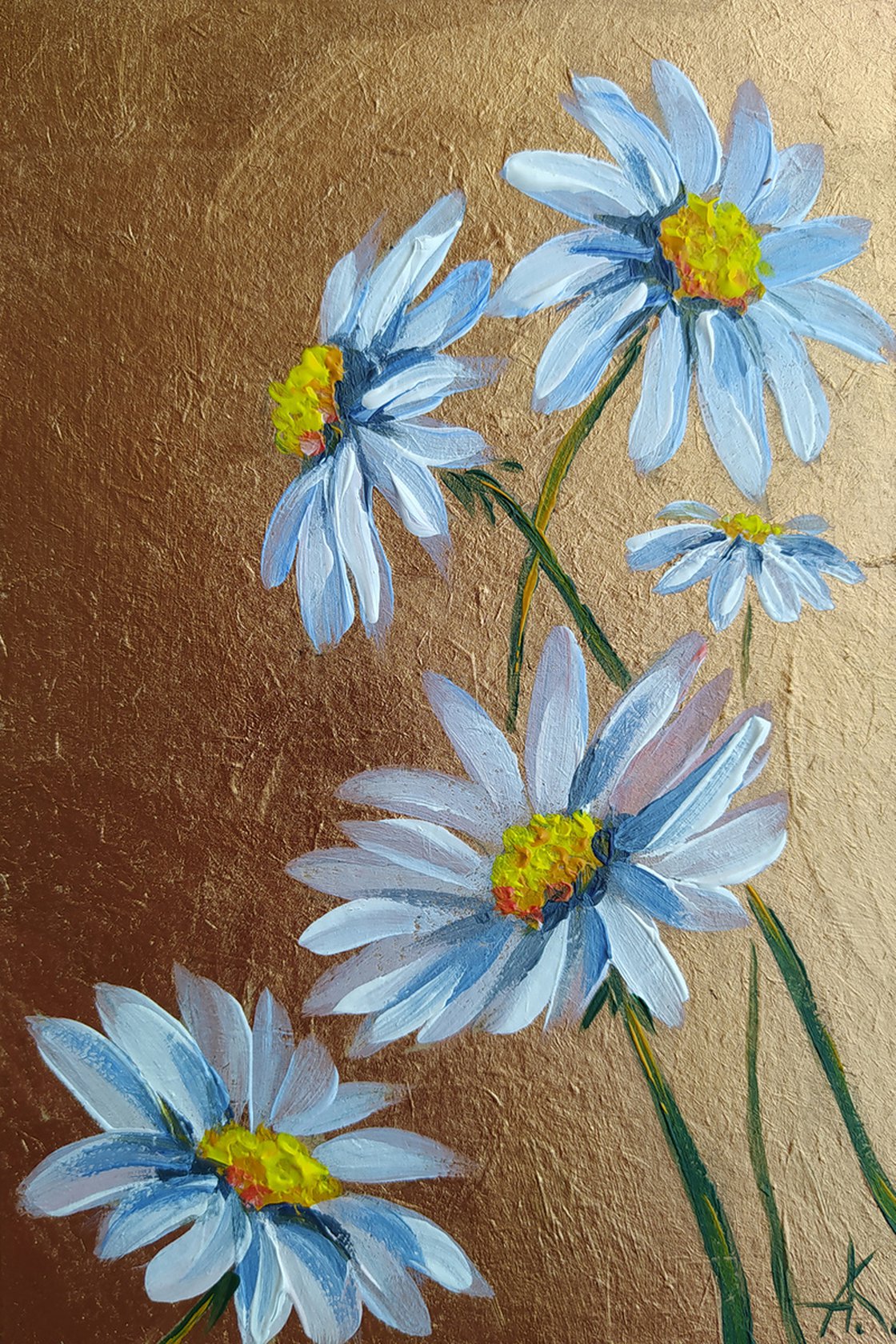This detailed painting appears to be created with oil paints, vertically oriented, and features five daisies with a distinctive texture. Each daisy has delicate blue petals with splashes of white, giving them a light blue hue, and vibrant yellow centers. The flowers are positioned with long, realistic green stems that intertwine and point in different directions, adding a sense of dynamism to the composition. The background transitions from a lighter beige on the right to a darker tan on the left, enhancing the contrast and depth of the scene. The paint is applied thickly, creating rich textures and capturing the light beautifully. Near the bottom right corner, the artist has signed the work, possibly with the initials 'AK.' Overall, the painting exudes a vibrant, yet serene atmosphere with its skillful use of color and texture.